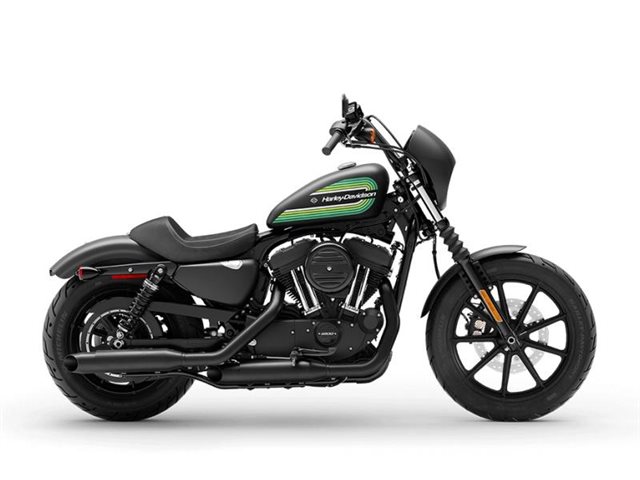This image depicts a sleek, all-black Harley Davidson motorcycle viewed from the side against a crisp white background. Notably, the traditional Harley Davidson logo is present, but it features unique green lines and stripes of yellow and blue that gracefully arch around the emblem, giving it an uncharacteristic appearance. The motorcycle boasts a shiny finish, with visible details such as a seat, handlebars equipped with a brake system, and two wheels—one at the front and a rear tire surrounded by various mechanical components. While the front tire is exposed, the rear tire is notably more intricate in design. A subtle green hue permeates the image, adding an extra layer of distinctiveness. The motorcycle's shadow is the only other element contrasting the white background, emphasizing the bike's glossy and pristine design. This image, with its clear and polished presentation, suggests it could be a stock photo ideal for online advertisements.